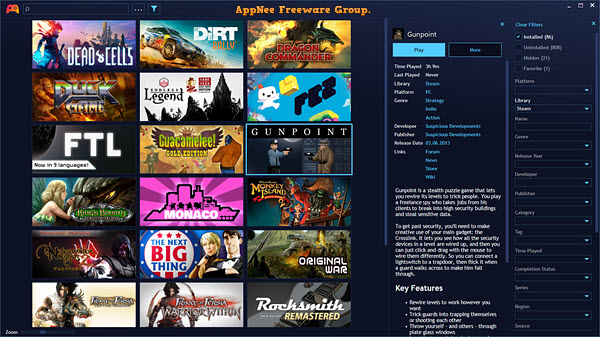This digital image showcases a list from the Apnea Freeware Group, prominently displayed at the top. On the left side, several thumbnails are visible, each representing different titles. The first thumbnail is for "Dead Cells," featuring an animated character with vibrant red hair. Adjacent to it is "Dirt Rally," displaying a vehicle navigating through a dirt track. Next is "Francis Commander," depicted with an intricate illustration of a dragon. Following that is "Duck Grind," with a visual of a gorilla. "Pez" features a small, white cartoon character. The lineup continues with "FTL" and "Guacamelee Gold Edition." A thumbnail for "Gunpoint" shows an officer aiming a gun at a detective. Further down is "Monaco," followed by "The Next Big Thing," "Original War," "Rocksmith Remastered," and "Warrior Within." At the bottom of the list are a play button and a more button, inviting interaction.